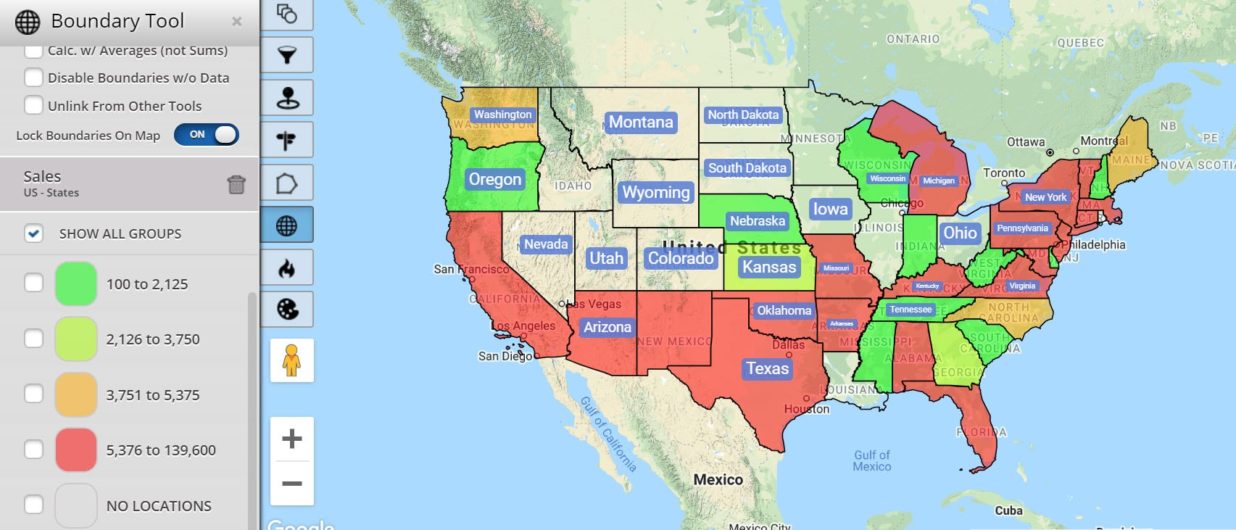A detailed descriptive caption for the given image could be:

---

The image is a screenshot displaying a two-column interface. On the left, the creamy light brown sidebar includes various settings related to data visualization. The top section is titled "Boundary Tool," featuring options like "Calculate with averages, not sums" (unchecked), "Disable boundaries without data" (unchecked), "Unlink from other data" (unchecked), and a toggle switch for "Lock boundaries on map," which is activated.

Below these settings, under the section named "Sales, US States," there are several checkbox options indicating data ranges for color-coding states on the map. These ranges are:
- "100 to 2125" (green)
- "2126 to 3750" (yellow)
- "3751 to 5375" (orange)
- "5376 to 139,600" (red)

All these options are checked.

The right column features a map of the United States where states are color-coded according to the aforementioned ranges. For instance, states such as New York, Pennsylvania, Virginia, Michigan, Oklahoma, Texas, and Arizona are highlighted in red, indicating the highest data range (5376 to 139,600). In contrast, states like Oregon, Nebraska, Wisconsin, Tennessee, Indiana, and West Virginia are marked in green, representing the lowest data range (100 to 2125).

This visualization helps in analyzing data distribution across different states using color segmentation for easier interpretation.